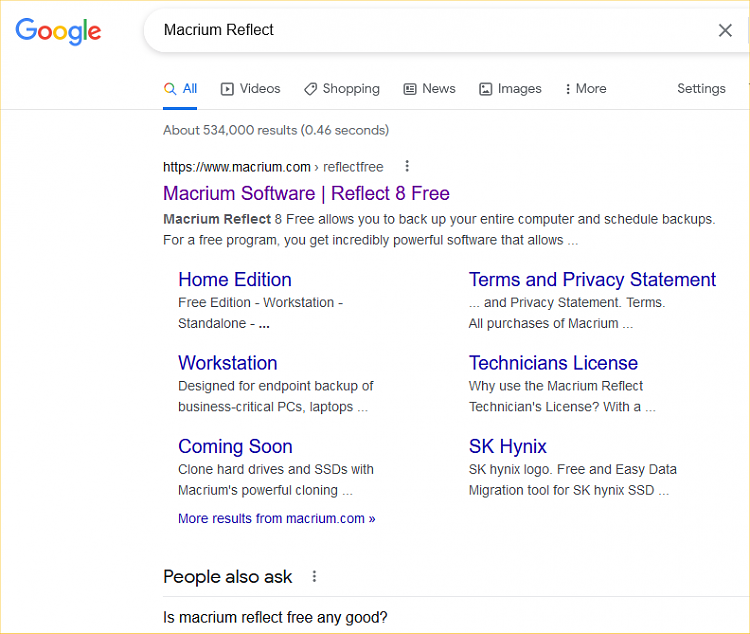This is an extremely detailed and cleaned-up caption for the described image:

---

The screenshot showcases a Google search result page featuring the classic Google logo in the top left corner with its iconic colors: blue 'G', red 'o', yellow 'o', blue 'g', green 'l', and red 'e'. To the right of the logo, a prominent search bar spans across to the right edge of the page. Inputted in the search bar is the query: "Macrium Reflect". Adjacent to the search bar on the far right is a small 'X' icon, framed by a thin gray border against a white background.

Below this is the search navigation bar, starting slightly off to the left. The first option in blue text reads "All" and is underlined, indicating the currently selected category. Following this are several other navigation options in black text, each accompanied by corresponding icons on their left: "Videos", "Shopping", "News", "Images", and "More". On the far right, without an icon, is the "Settings" option.

Underneath the navigation bar, Google has listed the search results, starting with the information about the number of results and the time taken to fetch them. The first search result shows the link to Macrium Reflect's website, displayed as:

`https://www.macrium.com > Reflect Free`

This is followed by a description in purple text: "Macrium Software - Reflect 8 Free". Below this title are two lines of black text describing the software. Further details are organized under the headings 'Home Edition', 'Workstation', and 'Coming Soon', each followed by more descriptive text and links. To the right of these headings are terms like 'Privacy Statement' and options such as 'Technician’s License' and 'SK Hynix', each hyperlinking to detailed information. Beneath 'Coming Soon', there's an additional link: "More results from macrium.com".

Further down, a section titled "People also ask" is presented in black text, with a sample question displayed: "Is Macrium Reflect Free any good?"

---

This detailed caption captures the structure and content of the Google search results page as described.